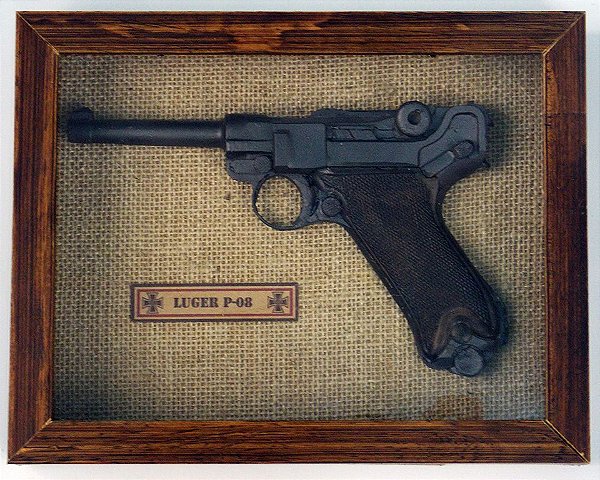The image portrays a black antique Luger P-08 pistol presented as a display or collector's item within a horizontal, rectangular, dark red wooden frame resembling cherry wood. The frame's matting is made of a brown and beige material, reminiscent of a burlap sack, giving it a rustic and aged appearance. The Luger P-08, primarily black with a textured grip, appears compact and battle-worn, with visible corrosion around the trigger assembly and the butt of the handle, as well as scuff marks on the frame and burlap backing. The barrel of the pistol points to the left, and it is accompanied by a rectangular placard bearing the text "Luger P-08" and adorned with iron crosses. The display piece looks well-used, suggesting it has likely been fired and bears the marks of time and usage.